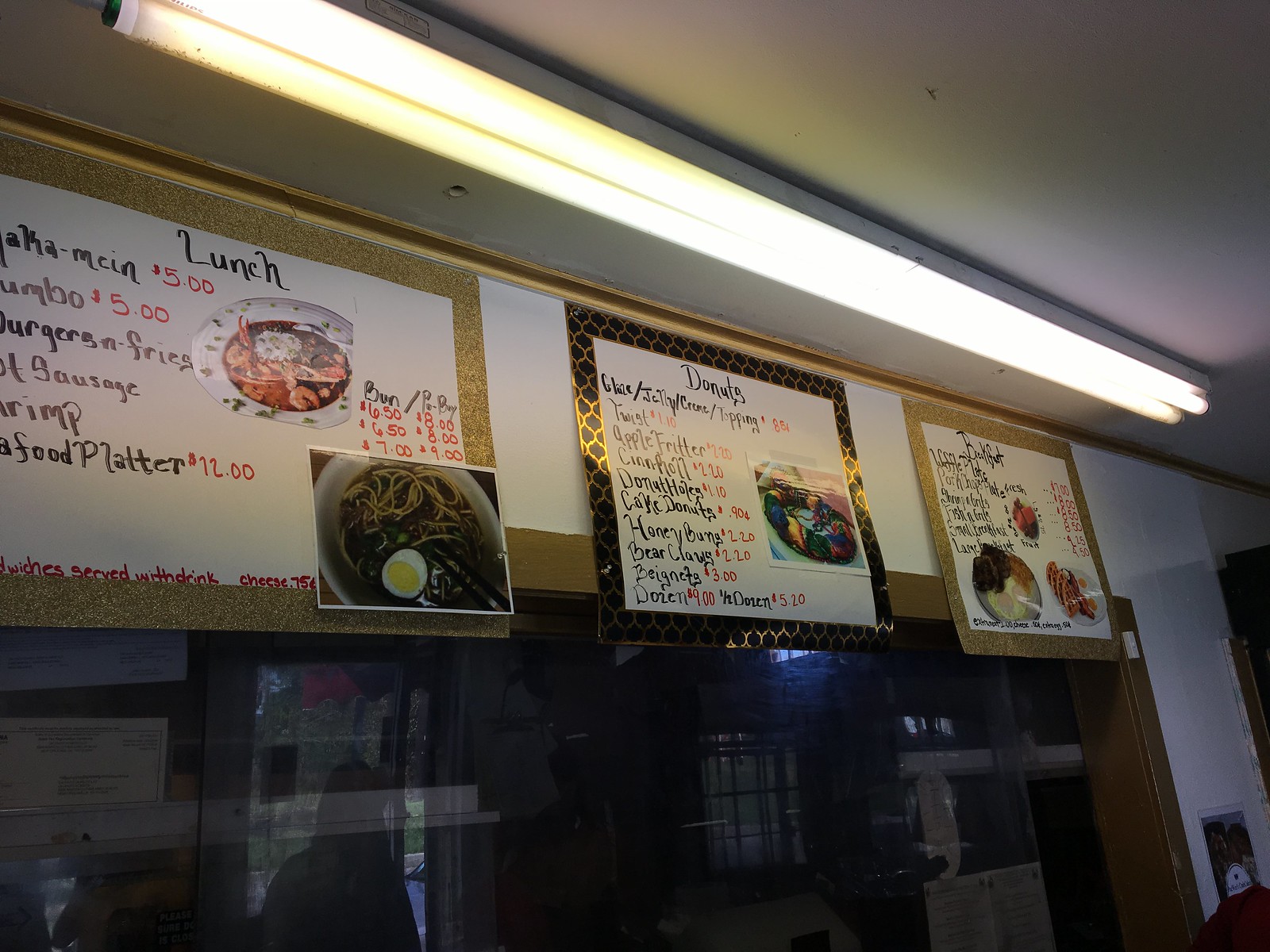This photo captures the interior of a rather dingy restaurant, focusing on three overhead menus positioned above a food counter. Each menu appears to represent different meal sections, possibly lunch, dinner, and an unidentified category, though their details are not fully legible. The menus are accompanied by two photographs of food items each, arranged in a square tabular format. Dominating the scene is a massive fluorescent light fixture suspended above the menus, casting a stark, clinical light on the surroundings. Below the overhead menus, the counter features clear transparent barriers with a hint of black framing, adding to the overall uninviting ambiance of the establishment. The image is taken at a slight angle, giving a skewed perspective of the setup.